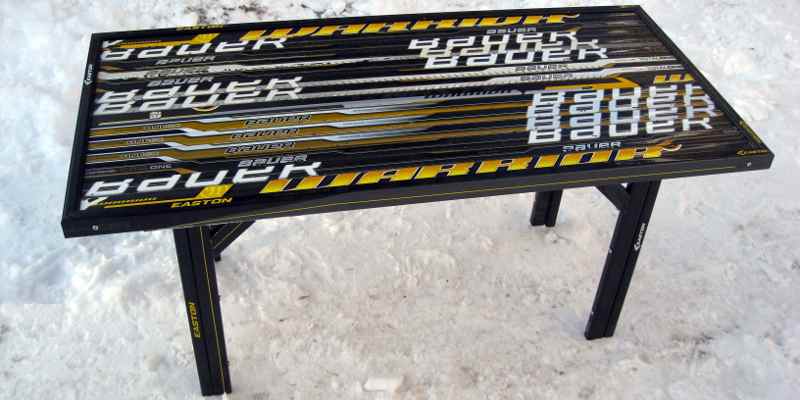The image depicts a small, portable table set outdoors on a packed snowy ground. The table, which appears to be made of metal, has four foldable black legs with branding on them. The most prominent branding includes the words “Easton” and possibly “Bauer” or “Bowa,” although the latter is less clear due to tapered lettering. The tabletop is black with additional white and yellow lettering, potentially referring to the brands mentioned. Despite being placed in snow, it is not immediately clear what specific purpose, if any, the table serves beyond its apparent promotional logos. The scene is captured during daylight, accentuating the stark contrast between the dark table and the bright snow.